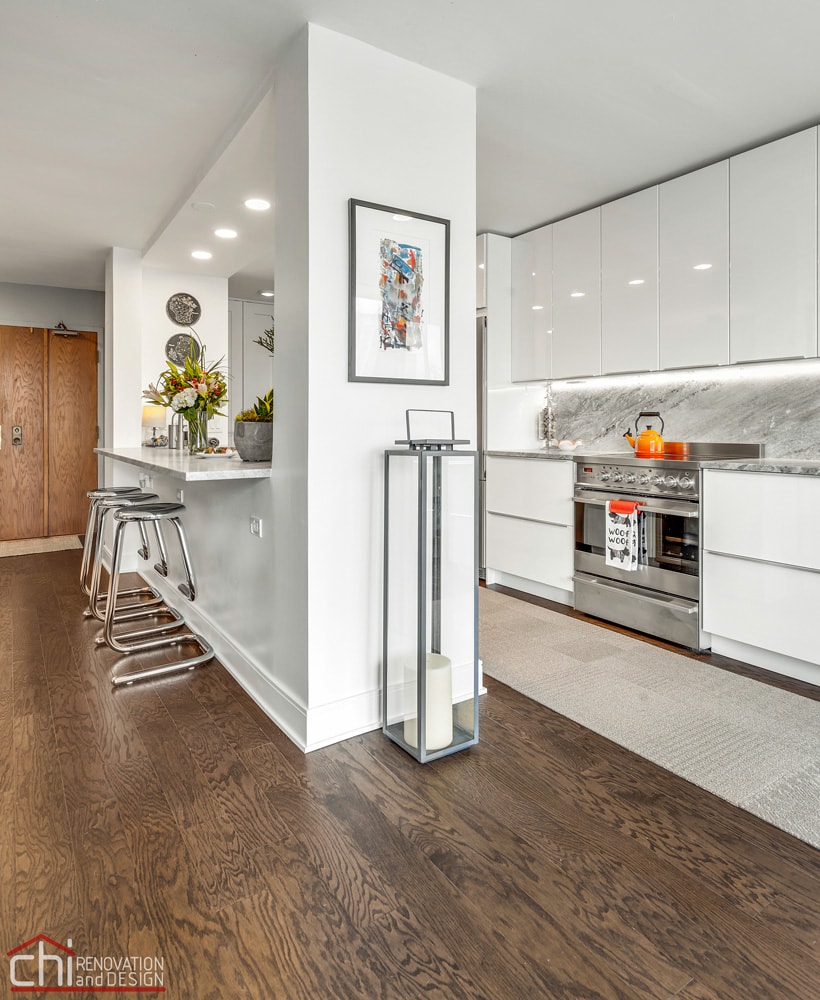The image depicts a stylish, well-presented kitchen and adjoining living space within a home, resembling a layout featured in upscale home decoration magazines. The kitchen area on the right side of the image showcases a large, stainless steel chef-style stove with an orange teapot perched on top. Surrounding the stove are white cabinets equipped with gray marble countertops and a matching gray marble backsplash. The floor directly in front of the stove is thin and gray, transitioning to dark brown wood flooring that extends throughout the room.

Adjacent to the kitchen is an island-style bar countertop with a white granite surface, illuminated by three spotlights from above. The countertop features two flower vases and is accompanied by three metallic silver bar stools placed to the left, providing a casual seating arrangement that opens into the kitchen area. The walls are painted white, matching the white ceiling, creating a bright and cohesive atmosphere.

Further left, the room displays brown cabinets on the far wall and a closed brown door. Notably, a small painted artwork is fixed on the central wall, enhancing the room's aesthetic. In the bottom left corner of the image, there's a logo with "CHI" in white letters, a red triangle above it, and a red line extending beneath it, branded with the text "Renovation and Design."